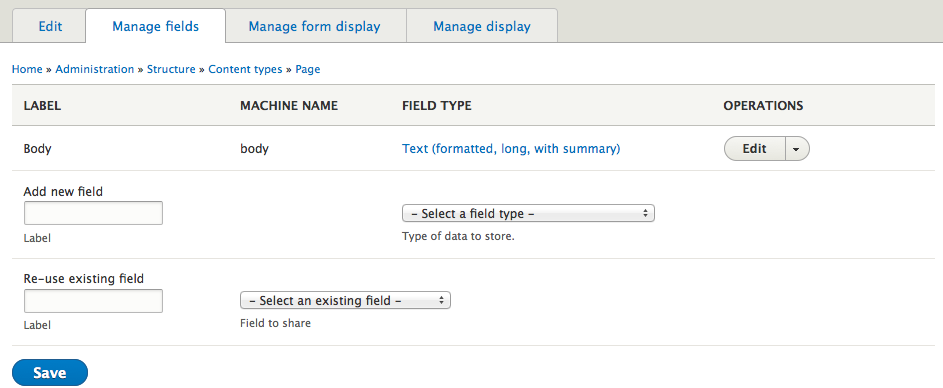The image captures a screenshot of a computer screen displaying a web browser with multiple open tabs. The user is currently viewing the second tab titled "Manage Fields." The other visible tabs include "Edit," "Manage Form Display," and "Manage Display," all labeled in blue text.

At the top of the "Manage Fields" area, there is a breadcrumb navigation path in blue that reads: "Home > Administration > Structure > Content types > Page." Below this is a section with a gray background and black text featuring multiple columns. The labels for these columns, from left to right, are "Label," "Machine Name," "Field Type," and "Operations."

The first row under "Label" contains the text "Body," which is also repeated in the "Machine Name" column. The "Field Type" column indicates "Text (formatted, long, with summary)." Located in the "Operations" column is an "Edit" button with an associated drop-down menu.

At the bottom of the screen, there are options for "Add new field," "Reuse existing field," and a blue "Save" button.